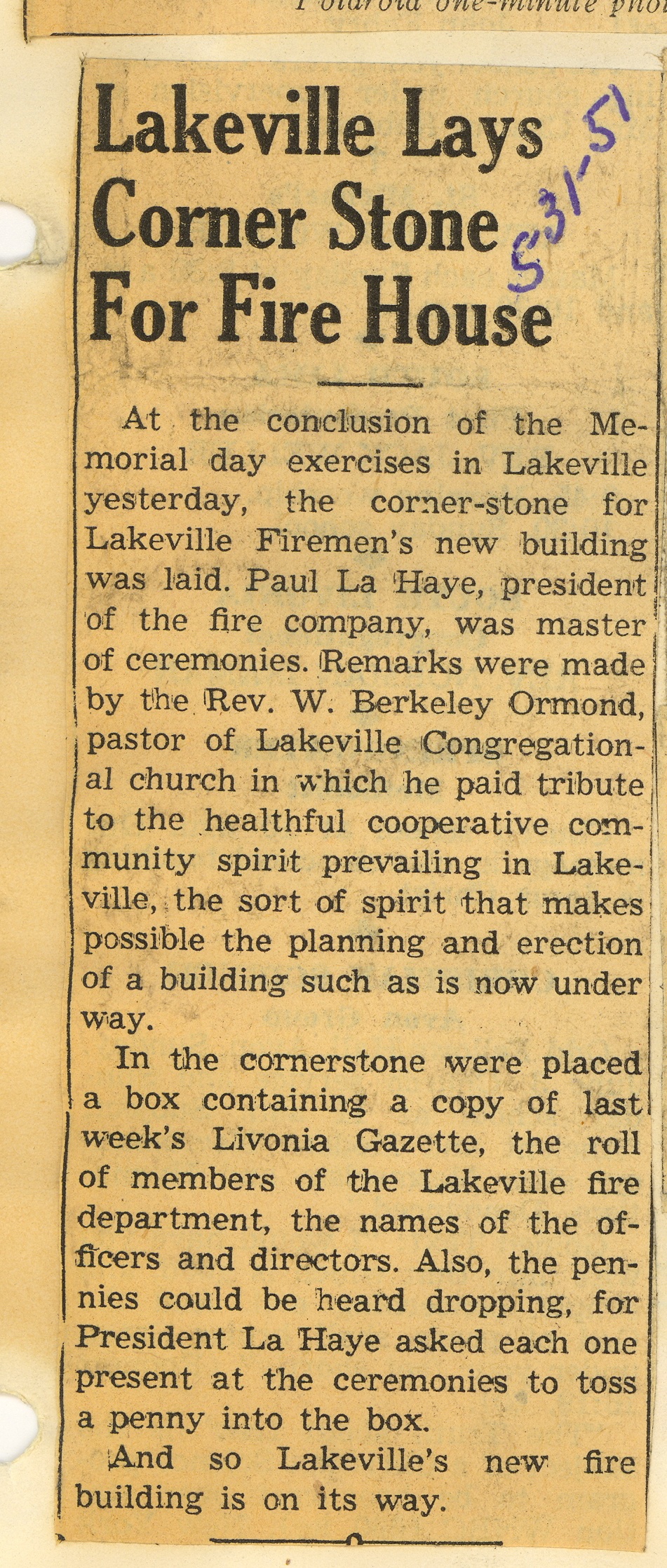This image features a scanned, yellowed newspaper clipping from May 31, 1951, annotated in ink with the date "5-31-51" at the top. The article, titled "Lakeville Lays Cornerstone for Firehouse," describes the ceremony held at the conclusion of the Memorial Day exercises in Lakeville. The clipping, likely preserved in a scrapbook as indicated by the visible three-ring hole punches along its edges, details the laying of the cornerstone for the new Lakeville Firemen’s building. Paul LaHaye, president of the fire company, served as master of ceremonies, while Reverend W. Berkeley Ormond, pastor of Lakeville Congregational Church, delivered remarks celebrating the community’s cooperative spirit. The cornerstone ceremony included placing a time capsule containing a copy of the previous week's Livonia Gazette, a roster of fire department members, the names of officers and directors, and pennies contributed by attendees at LaHaye's request. The faded clipping, set against a tan background, captures a historical moment with its black-and-white print now tinged with a distinctive orangish hue.